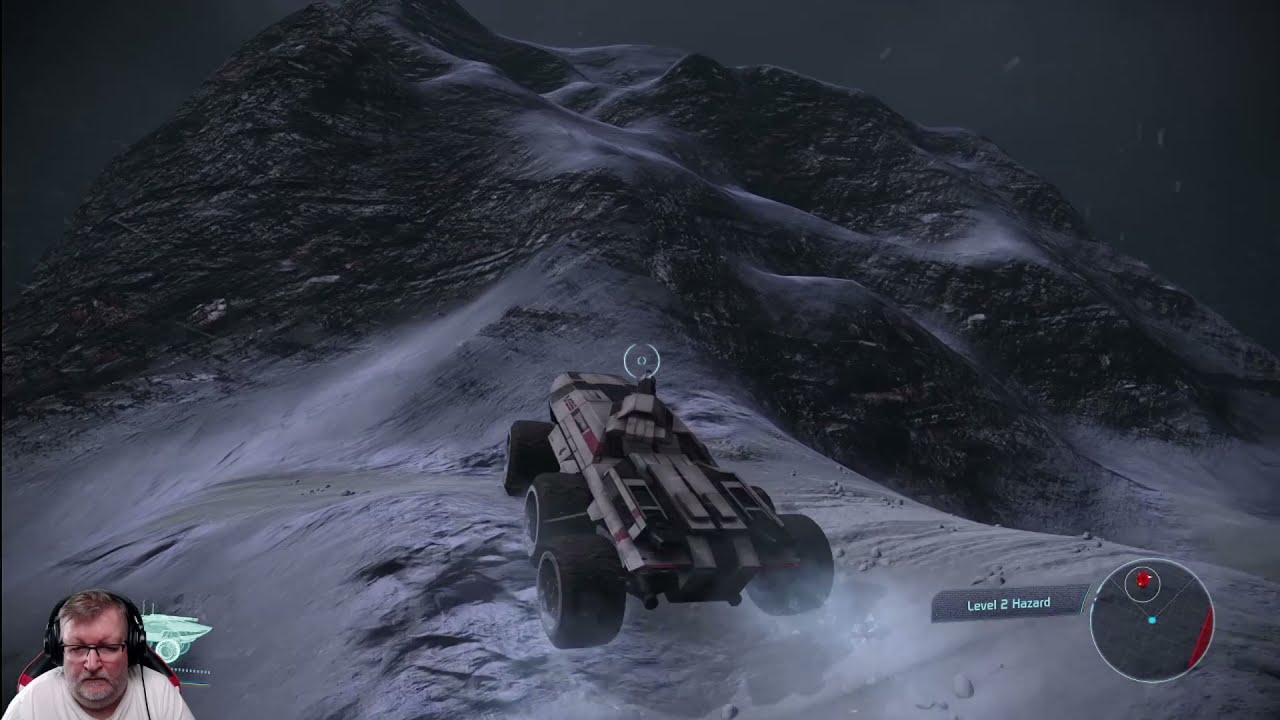The image captures a screenshot of a live-streamed video game session. In the bottom left corner, an elderly white man, approximately 50 years old with gray hair, glasses, a slight gray beard, and a white t-shirt, is shown sitting in a gaming chair. He is wearing black headphones and is actively engaged in the game. The main screen displays a nighttime mountainous scene, with a white, six-wheeled armored vehicle, equipped with a roof gun, traversing a snowy, dust-covered hill. The terrain features a prominent mountain in the middle. In the bottom right corner, a navigation map labeled "Level 2 Hazard" indicates the current game difficulty.